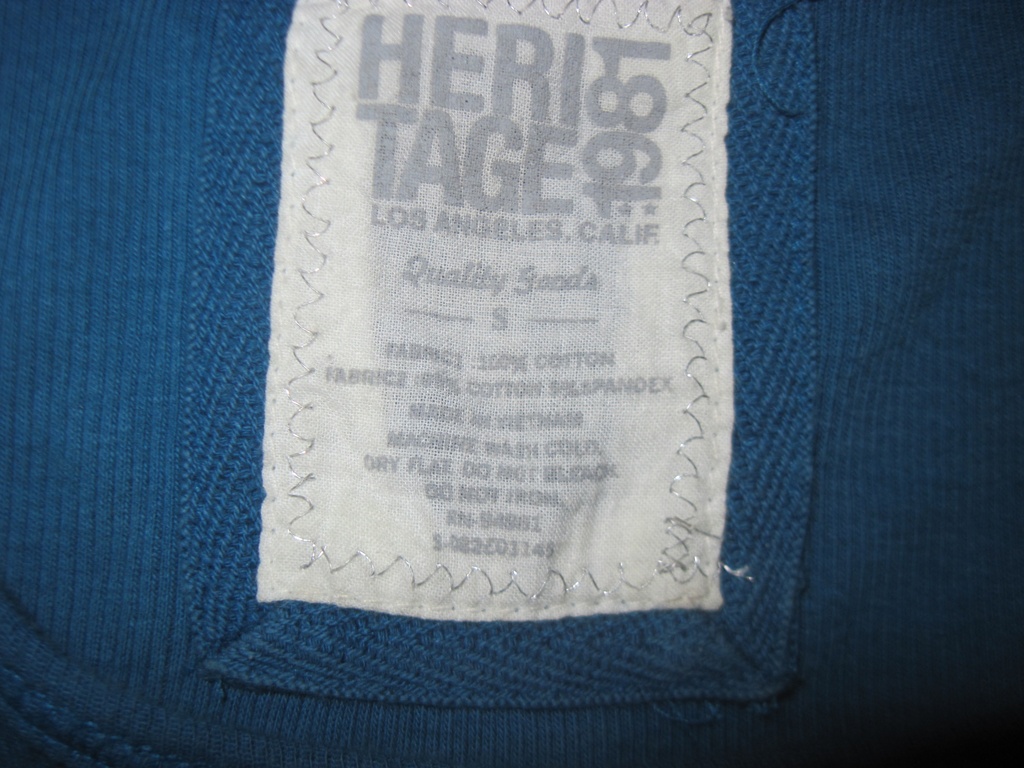This close-up, color photograph prominently features a rectangular, fabric label attached to a piece of dark blue, net-like fabric. The fabric label, bordered by a zigzag stitching, occupies most of the height and about half the width of the image. Surrounding the label are visible seams in the same blue fabric, creating a framed effect.

The label itself appears white or very pale grey, possibly with some staining or shadows giving it a slight discoloration. At the top of the label, in grey text, is "H-E-R-I," placed above the letters "T-A-G-E," forming the word "heritage." Rotated 90 degrees to the left, the number "1981" is inscribed vertically. 

Horizontally aligned below this are the words "Los Angeles, California." Further down, the text "quality goods" is written in cursive. The label then indicates the size as "S," likely denoting small. The fabric composition is stated as 100% cotton, although there are some variations and additional materials mentioned, including a possible percentage of spandex.

Further details become increasingly hard to decipher due to fading. However, care instructions such as "machine wash cold," "dry flat," "do not bleach," and "do not iron" are visible. There is also some identifying information at the bottom, including an R and S number along with other numbers and characters, though these remain largely unreadable due to the photograph’s detail level. This label, though highly zoomed in, suggests it belongs to a small blue clothing item, possibly made in Vietnam.